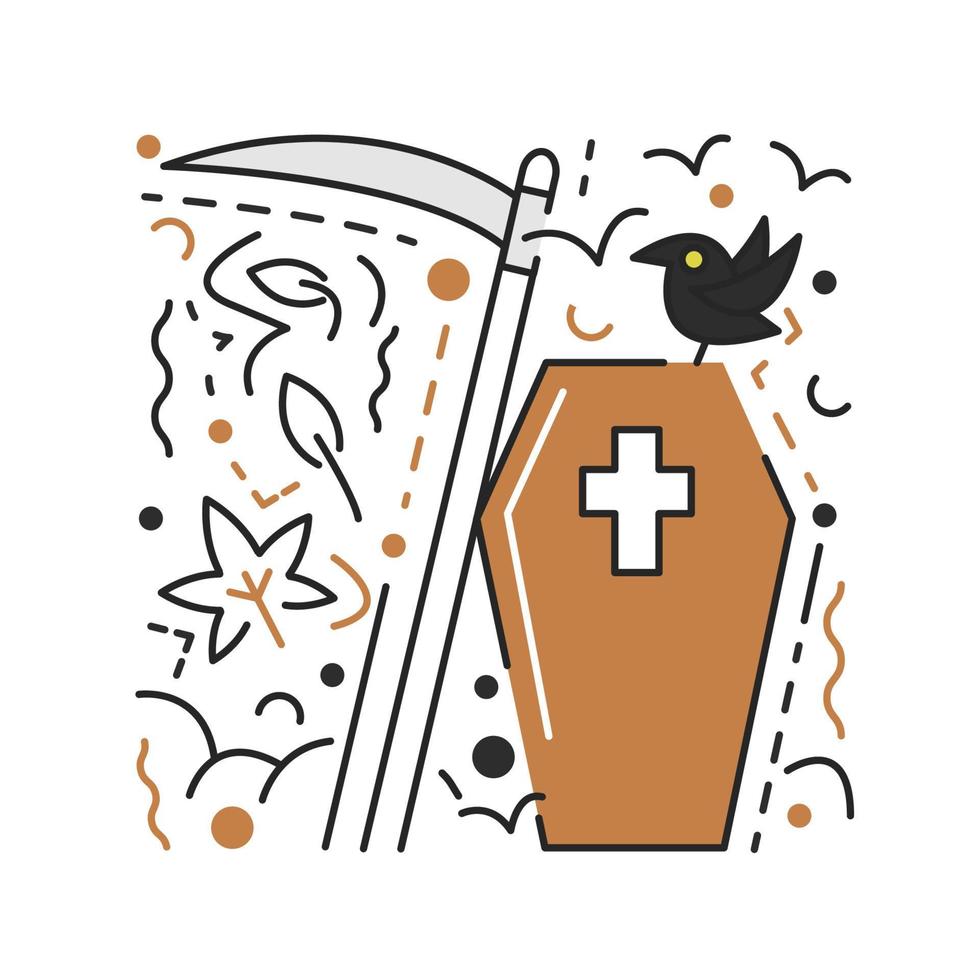This whimsical yet morbid piece of artwork depicts a vertically standing, tan coffin with a large prominent white cross bordered in black on its front. The coffin, outlined with thin black lines, has a mysterious, almost solemn appearance. Atop the coffin perches a small black crow with a striking yellow eye. Leaning against the left side of the coffin is a large scepter with a menacing silver blade, reminiscent of a sickle left by the figure of Death. The scene is intricately adorned with simple black line drawings of leaves and various abstract elements, including squiggly lines, dots, broken dashed lines, and even faint impressions of distant crows, adding to the haunting and detailed nature of the composition.